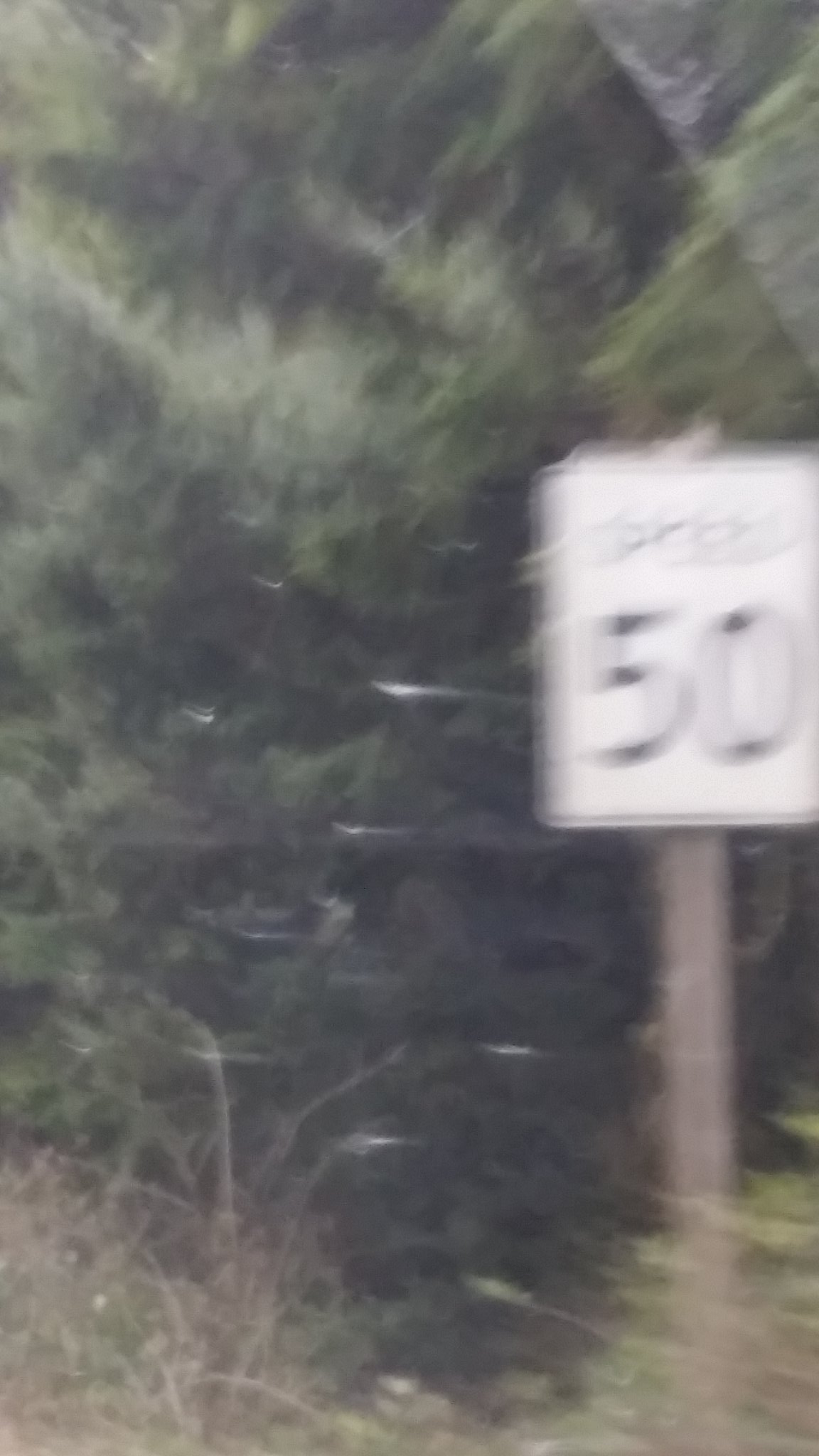In this extremely blurry and grainy image, we see a white speed limit sign positioned vertically along the side of a road, possibly attached to either a wooden or metal post. The sign, featuring a black trim, clearly displays "SPEED" in capital letters with the number "50" directly beneath it. This image appears to have been taken from inside a moving vehicle, as evidenced by the pronounced motion blur and possible streaks on the windshield.

In the background, a densely packed forest of pine trees quickly darkens, potentially blocking out much of the sunlight and creating a shadowy area in the middle of the image. The foreground is cluttered with various plants, weeds, and bushes, adding to the overall sense of a rural or off-road setting. There are indistinct white spots throughout the image, which could be either floating particles from plants or insects in the air. Additionally, there is a noticeable glare and reflection, suggesting light is coming from the top right corner, further adding to the difficulty of distinguishing specific details. The positioning of the sign aligns with the far-right edge of the photo, and the shot seems to be captured in a way that the center of the sign is just above the halfway point of the frame.